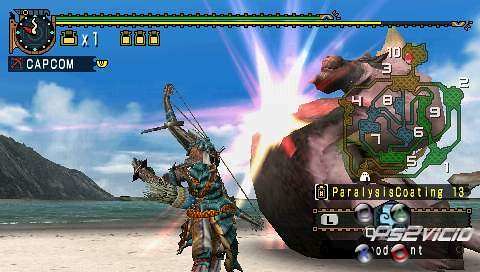In this screenshot from a Capcom video game, two characters are engaged in a heated battle. At the top of the screen, a green energy bar denotes their health levels. The backdrop features a blue sky with flames emanating from one of the characters. Sparks fly as the character attempts to defeat his opponent. In the lower left-hand corner, a clock reads "Times 1" beneath the Capcom logo. The scene is set on a sandy beach with an ocean view, flanked by mountains on the side. A colossal, blob-like creature with brownish hair dominates the right side of the screen. This creature is labeled with "Paralysis Coding PS2" around its edges. One of the combatants is equipped with a bow and arrow and is dressed in green attire.